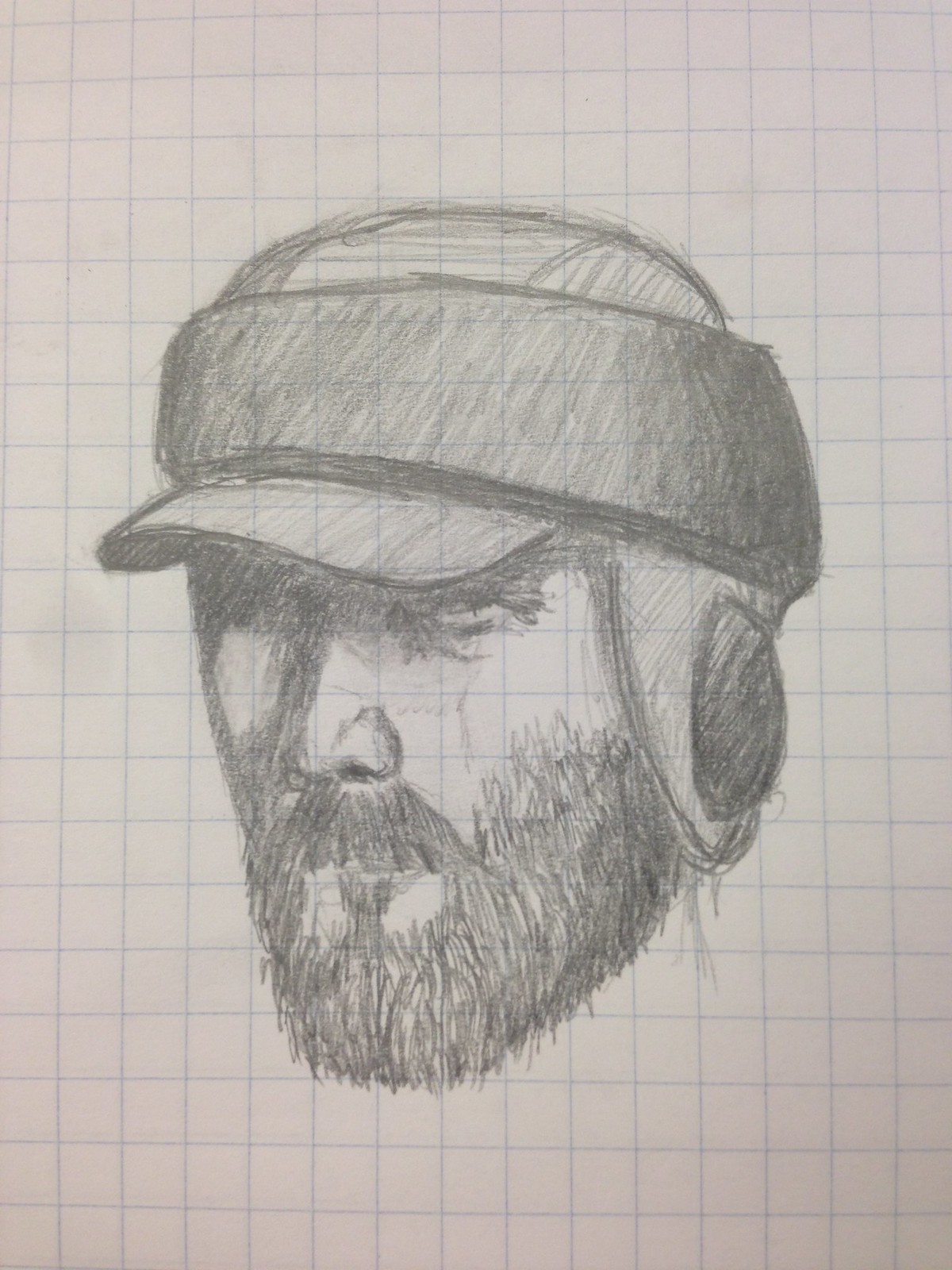This detailed graphite pencil sketch, drawn on graph paper with faint blue gridlines, focuses solely on the head of a bearded man. The man is depicted wearing a winter cap with ear flaps that cover his ears, creating a sense of seasonal cold. A headband, which might be part of the cap, wraps over the visor, contributing to darker shaded areas around the man's head. His beard is full yet trimmed to a shorter length, connecting with a short mustache under his lip to form a goatee. The man's eyes are obscured by the shadow cast by the cap's rim, enhancing his rugged look. His pointed nose and a pronounced frown give him a somewhat menacing expression. The entire sketch is strikingly detailed with careful directional shading, adding depth and texture to the monochromatic black-and-white drawing.